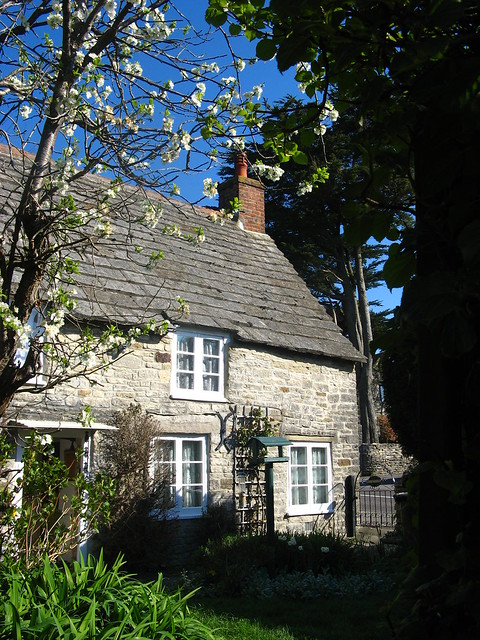In this image, there is a quaint, older-looking cottage made of gray stone with a darker gray, tiled roof. The house features a prominent red brick chimney. The sky is a clear, baby blue, adding a serene backdrop to the scene. In front of the house, there is a flowering tree with white blossoms, likely a dogwood, surrounded by green grass and foliage. The cottage has white-trimmed windows - three of which are stacked in a triangular formation on the right side - and a largely obscured door that appears to be either red or brown. Additionally, there is a large, shaded tree to the right of the house, casting a dark shadow over that side of the image. The foreground includes a makeshift garden or pathway with branches on trellises and a bird feeder, adding to the house's charming appeal.